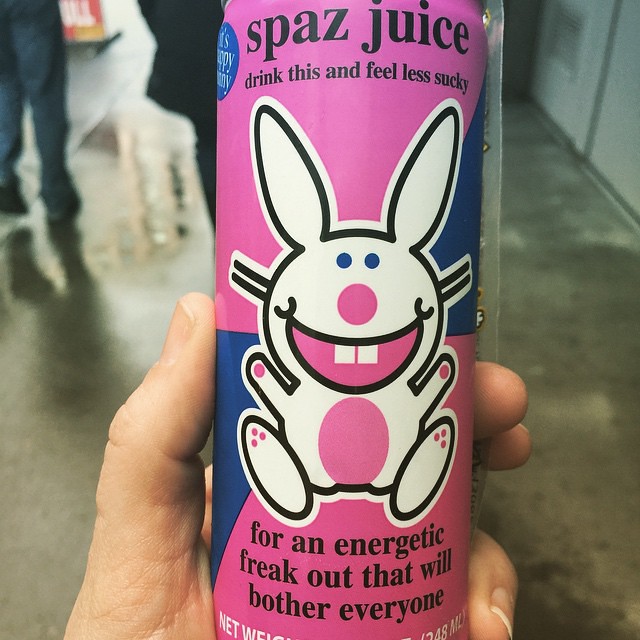The image showcases a can of SPAZ Juice held by a pale Caucasian left hand. The can features a prominent design with both pink and navy blue colors. At the top of the can, "SPAZ Juice" is written in black letters, followed by the slogan "Drink this and feel less sucky." Below the text, a cheerful white rabbit with a big pink smile, pink nose, pink belly, and paws outlined in black is depicted. The rabbit has navy blue eyes and appears lively against a navy blue diagonal stripe backdrop. Alongside the rabbit, the text "For an energetic freak-out that will bother everyone" is displayed on a pink background. The bottom text indicating the net weight is partially visible. A blue circle appears on the left side of the can, though its text is unreadable. The scene is set against a gray concrete floor with a wall to the right, and other people are visible seated in the background.